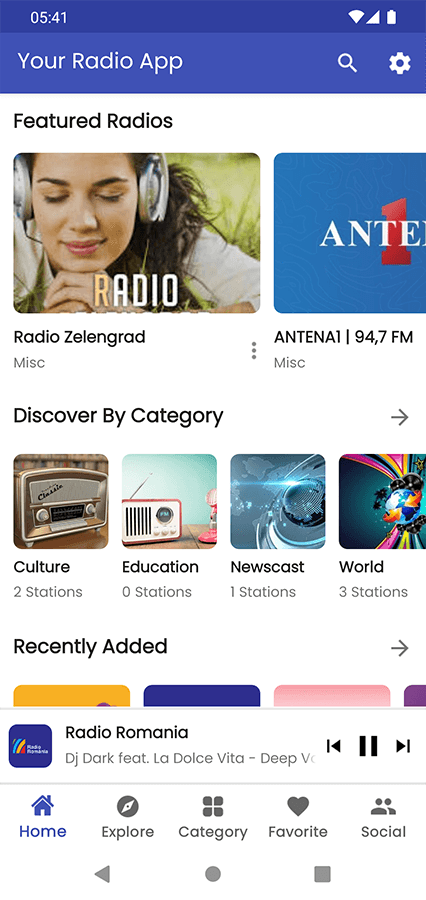The image displays a radio app with a blue-themed interface. At the top, there is a blue banner with the text "Your Radio App" in white letters. Adjacent to the text are icons of a magnifying glass, symbolizing search, and a gear, indicating settings. Above these elements are icons for Wi-Fi, battery life, and signal strength.

Below the banner, the heading "Featured Radios" is written in black. The first image features a woman with her eyes closed, her hands resting under her chin, and she appears to be enjoying music with vintage silver headphones. She is surrounded by greenery, suggesting she is outdoors. The caption beneath her image reads "Radio Zealot Zealot Grade Miscellaneous."

Next to this, there is a blue box labeled "Antena 1 94.7," with a subtitle "Discovered by Category" and a right arrow to preview more options. Below this box, there are thumbnails for different radio categories: 'Old Radio' with two stations, 'Culture' with no stations, 'Education' with zero stations, 'News' with one station, and 'World' with three stations.

Further down, the text "Recently Added" is partially visible, followed by four icons and a right arrow. Currently playing is "Radio Romania," indicated by a pause button and track navigation buttons. Below this, the song "DJ Dark featuring La Dolce Vita" is displayed.

At the bottom of the screen, navigation icons for Home, Explore, Categories, Favorite, and Social functions are present, with Home currently selected.